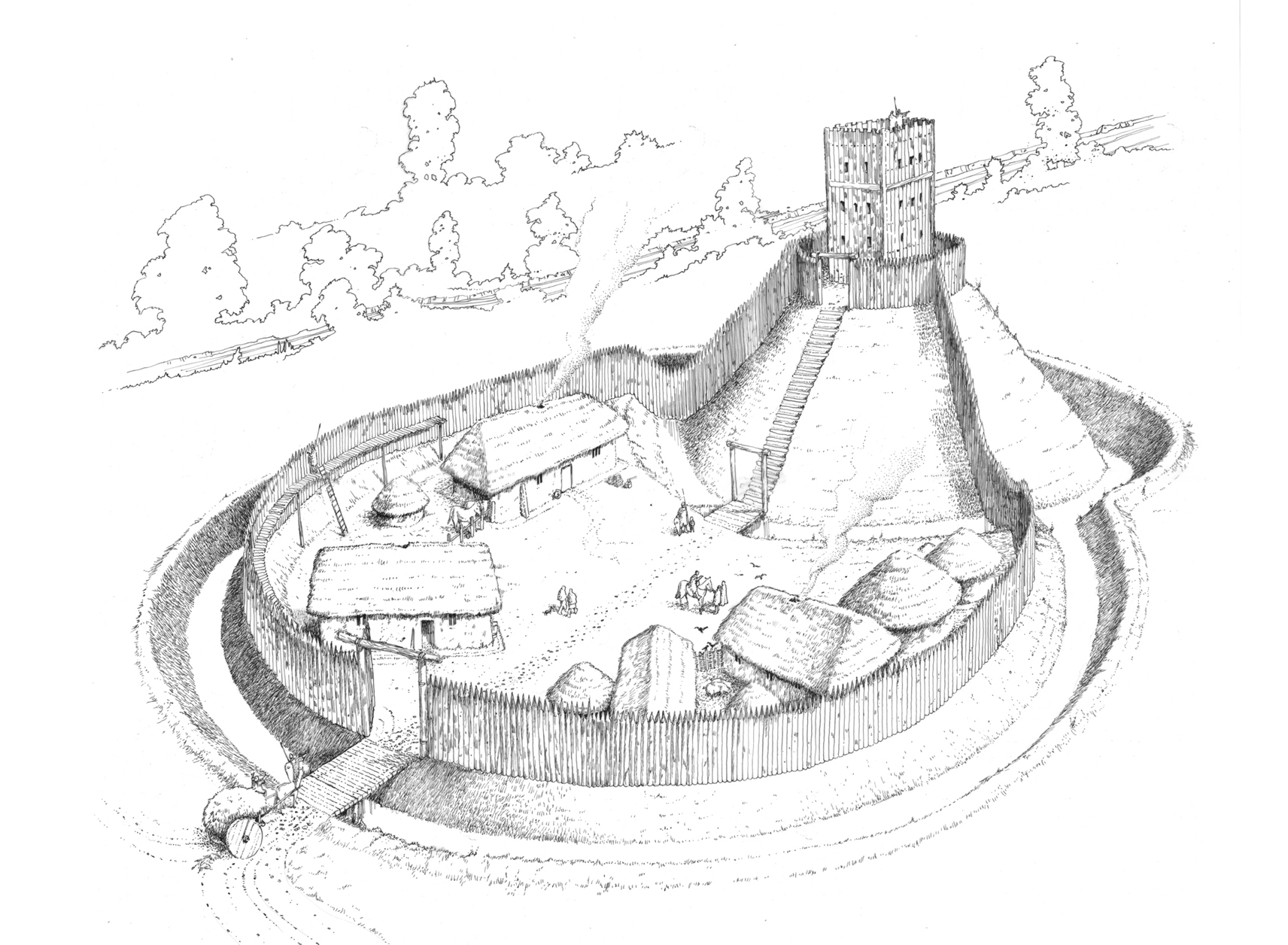The black-and-white drawing depicts an intricate, imagined fortress situated atop a conical hill. This three-story wooden fortress, resembling a castle, is fortified with sharp, tall pillar logs arranged in a circular fence designed to deter intruders. Access to the fort is secured by a wooden bridge spanning a surrounding water-filled moat. Within the fortified area, several wooden huts, including triangular longhouses and circular pyramid huts, are visible, each topped with hay roofs. The fort features a steep flight of stairs leading up to its elevated stronghold. In the background, lush trees and bushes add to the scene's depth, creating a vivid contrast to the manually detailed, clear depiction of the castle and village below.